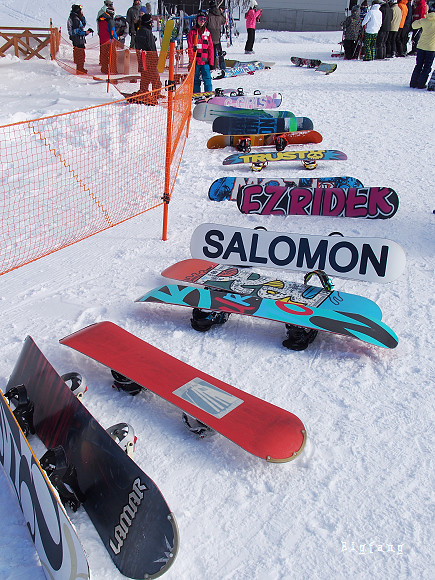This outdoor photograph captures a vibrant winter scene, featuring a collection of snowboards laid out on pristine, textured white snow. Dominating the image, these snowboards curve along a boundary marked by an orange mesh fence, creating a visually striking focal point. Each snowboard in the lineup is uniquely designed, adorned with a variety of colorful graphics and branding. The array includes black, red, teal, and graffiti-styled boards, alongside a white Salomon board with black lettering and an EZ Rider board in red font on black with a white outline. Additional boards showcase themes of trust with a skull, and a myriad of colors like orange, blue, green, and pink. In the bottom right corner, the text "Big Fang" is prominently displayed in white, spiky lettering.

In the background, two groups of snowboarders and skiers, bundled in winter gear including hats, coats, and snowboarding glasses, are visible. They are positioned more distantly on the left and right sides of the photograph. The snowboards' detailed appearances and the lively winter atmosphere suggest a scene from a snowboarding rental area or promotional material for a snowboarding company.